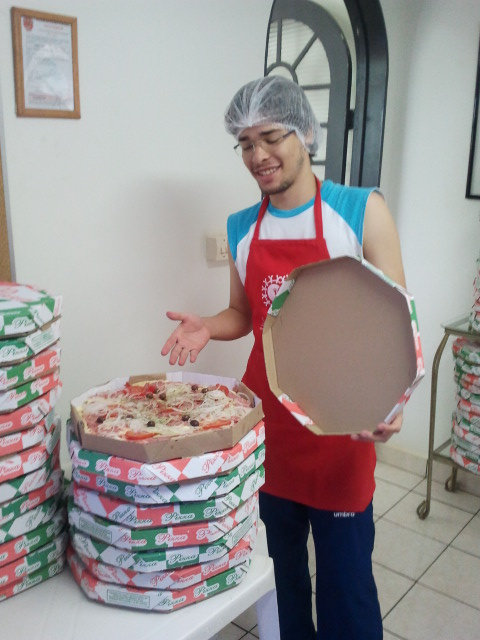The photograph captures a young man with slightly dark skin and black hair, wearing glasses and a white hairnet, inside a white-walled room with white tile flooring and dark grout. The man, who appears to be in his late teens to early 30s, sports a small goatee and a cheerful smile as he points at an open pizza box in front of him. He is dressed in a white and blue sleeveless athletic shirt, a red apron, and dark blue pants. The stack of five octagonal-shaped pizza boxes he's pointing to sits atop a white table, displaying a pizza with cheese, tomato slices, and black olives. Behind him, to the left, is another stack of approximately ten red, green, and white pizza boxes beside a metal cart with wheels. In the background, a black-framed door with glass panels and a grey archway enhances the room's decor, along with a white paper plaque featuring a red seal on the wall.